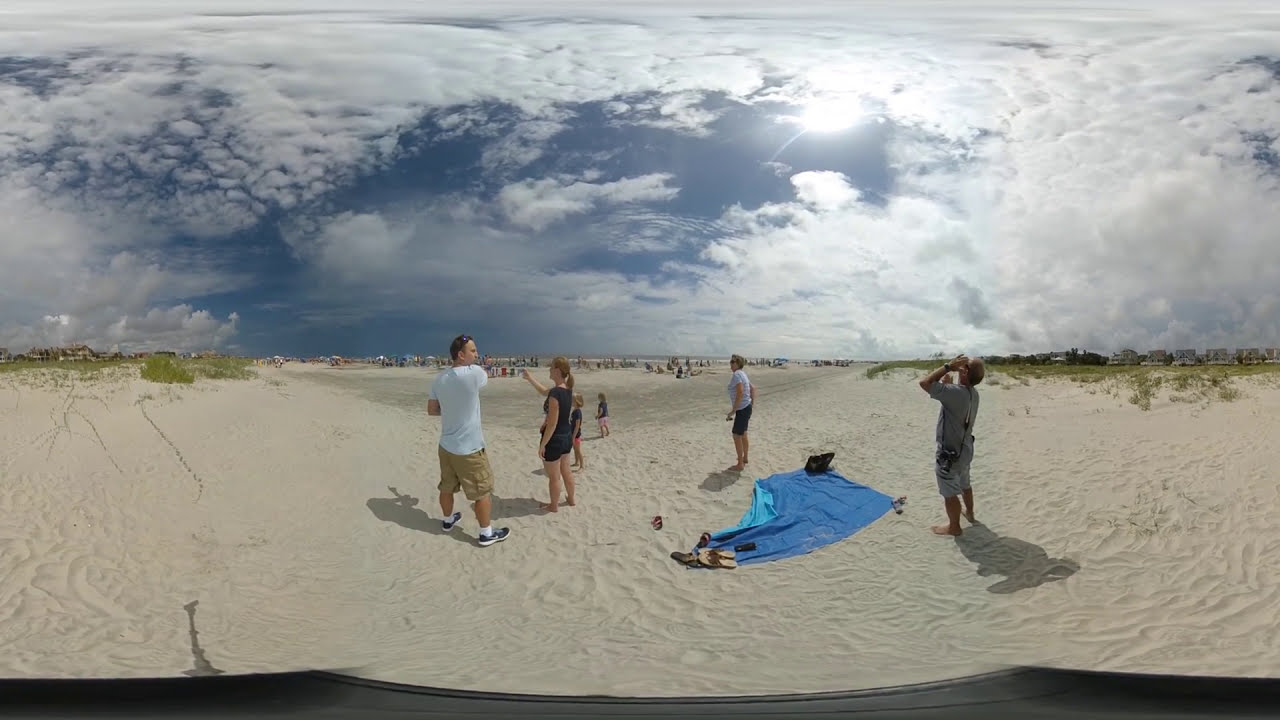A panoramic photograph captures a beach scene characterized by a vast expanse of light beige sand and a strikingly detailed sky, which occupies nearly half of the image and features an array of varied clouds. In the center of the frame are six individuals, including a man, a woman, and a couple of children, all dressed in shorts and t-shirts. They appear to be middle-aged, with a few kids around six years old, who seem to be looking in various directions—some at each other, some at the sky. A blue beach blanket lies on the sand near them, with one corner folded up, possibly due to the wind, and anchored down by sandals. Scattered around the blanket are flip-flops and other small items. Far in the background, numerous tiny figures are visible along the horizon, which would be closer to the waterline, although the water itself is not prominently displayed. On the far edges of the horizon, patches of green grass and a few buildings are faintly discernible. The sky is busy and vibrant, illuminated by the bright sun, and the entire image features some noticeable distortions, likely due to the panoramic technique or 360-degree imaging used.